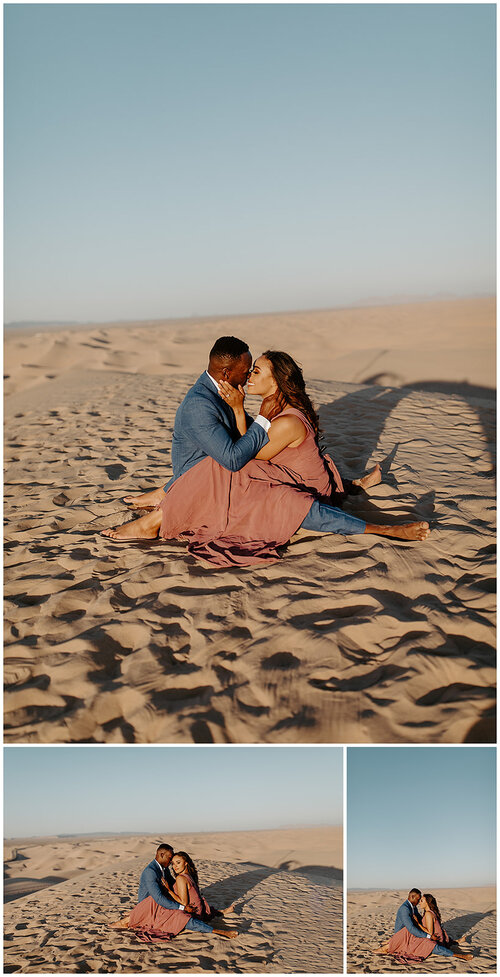This image is a rectangular montage, approximately six inches high and two to three inches wide, composed of three photographs depicting the same couple in an outdoor desert setting during the daytime. The top photograph, occupying 80% of the montage, measures about four inches high and showcases a blue sky that fades into a grayish haze near the horizon line. Below the sky lies a spread of finely coarse, light brown sand.

The couple, sitting in the sand, appears affectionate and possibly just married. The man, who looks to be of African descent with dark brown skin and short black hair, is dressed in a blue-gray suit jacket, a white collared shirt, and gray dress pants with no socks or shoes. He sits with his legs extended in front of him. The woman, who has light brown skin and dark brown hair, appears Middle Eastern and wears a pink sleeveless dress. She is positioned between the man's legs, facing left with her legs extended towards the same direction, and is also barefoot. In the top photo, the couple is engaged in an intimate moment, sitting close with the man’s hand on the woman's neck as they kiss.

Beneath the top photograph is a white horizontal border separating it from the two smaller photos. Each of the bottom photographs features the same couple in similar affectionate poses, maintaining the same sand and shadow details as the top image. On the left, the woman is looking towards the camera, and the man appears to be gazing at her. The rightmost photo, which is about half the size of the one on the left, shows the couple with their foreheads touching, gazing into each other's eyes, illustrating their close bond and affection for one another.